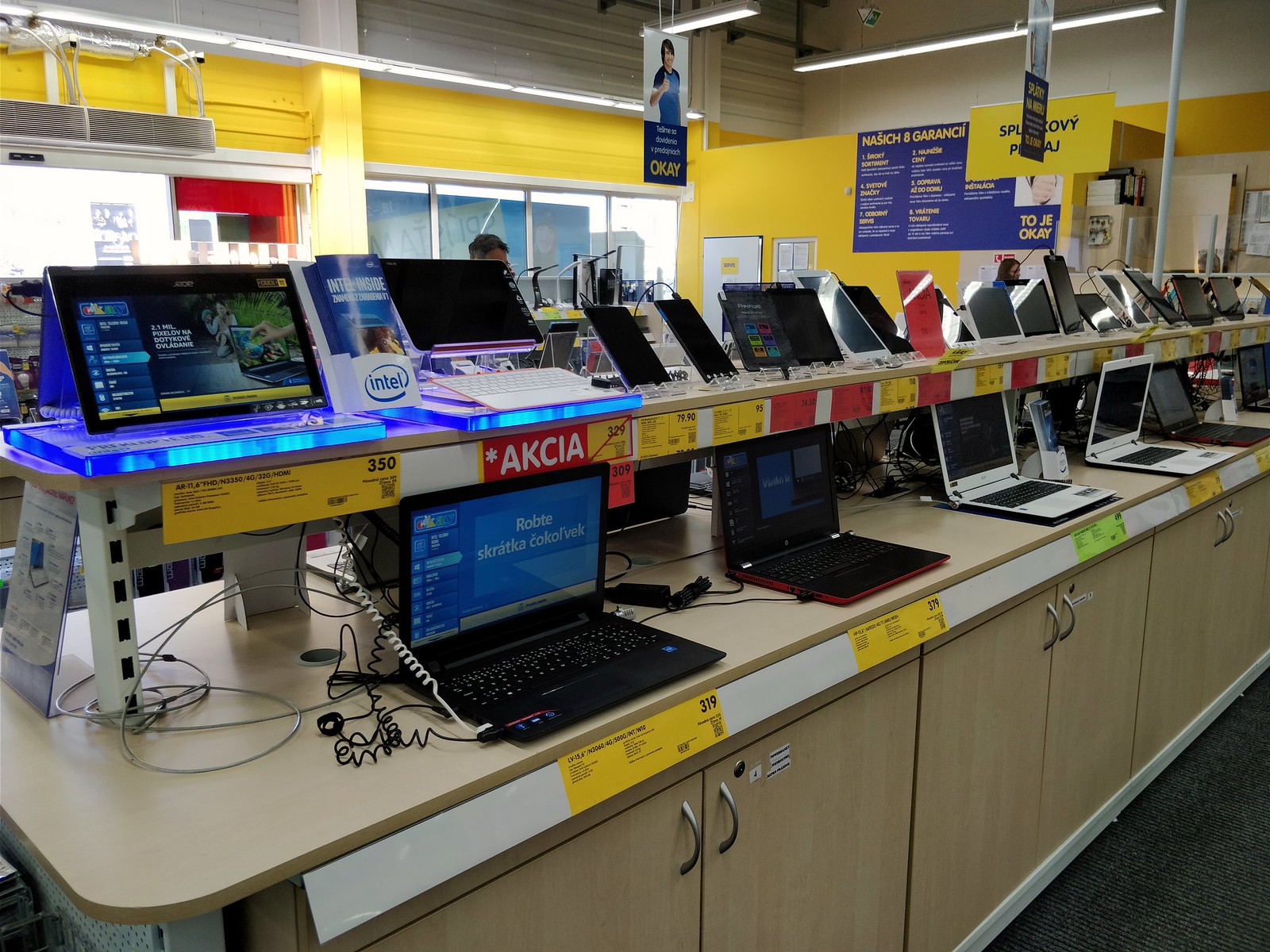The image depicts a computer display in an electronics store, likely Best Buy or Ikea, characterized by distinct blue and yellow signage featuring Swedish language accents. The setup consists of a two-tiered wooden cabinet and shelf system, showcasing an array of opened laptops of various colors, including black, white, and silver. The surfaces of the pale pine-colored cabinets support both laptops and some smartphones. Beneath each device, brightly colored price tags in yellow, green, and red offer product information. In the backdrop, the store walls are painted yellow, complemented by blue signage. Additional details include storage cabinets below the display shelves, a grey textured carpet in the bottom right corner, and part of a person's head visible behind the laptops slightly left of center, with another person near the right wall.